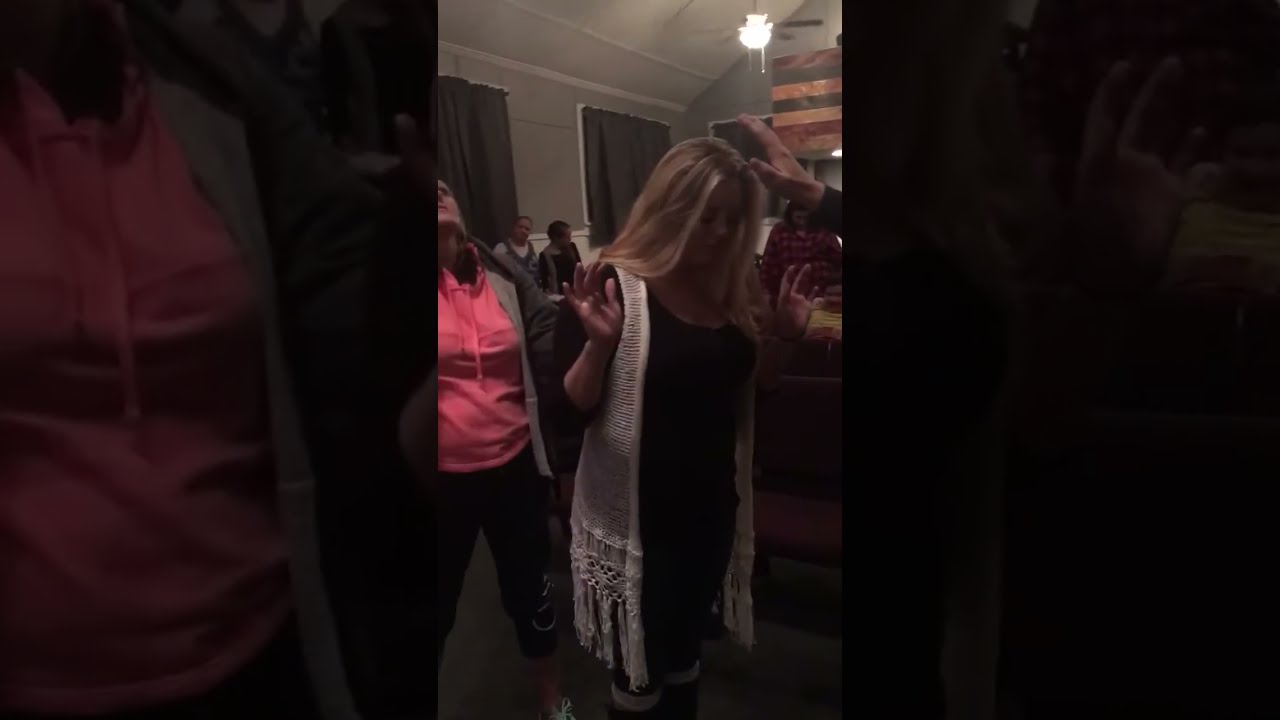In the image, the main focus is on two blonde women in the foreground of a dimly lit, large indoor venue, possibly an auditorium, with dark curtains and windows suggesting it’s suited for events. The woman on the left, who has blonde hair, is wearing a pink shirt layered with a grey jacket and a black coat over it, paired with black pants. She is looking up with a somewhat strange facial expression. To her right, the other blonde woman is dressed in a black and white outfit that includes a sheer, white, fringed vest over a black shirt or dress. She has her head tilted downward with one hand raised, possibly in a gesture of prayer or contemplation. In the background, a few men who appear to be in their 30s or 40s stand near what looks like an easel, adding depth to the scene. The overall lighting of the room is quite dark, contributing to the atmosphere of the setting.